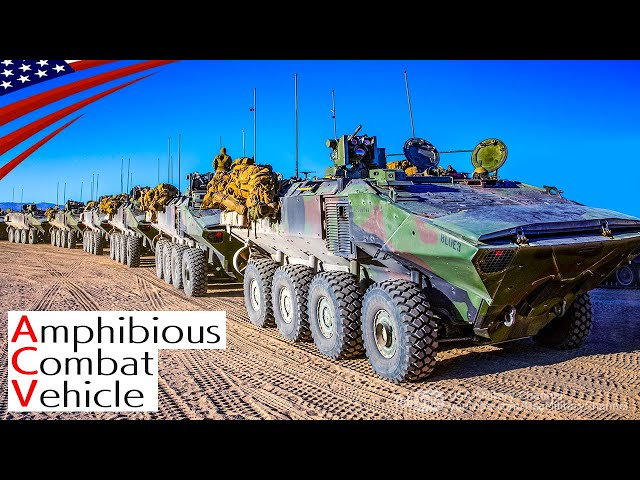The photograph depicts a line of six amphibious combat vehicles (ACVs) advancing across a sandy terrain under a bright blue sky. Each vehicle, painted in a camouflage pattern of green, red, and black, is equipped with four large wheels on each side and features mounted machine guns and multiple antennas. The vehicles have open hatches, with soldiers visible inside, and their design includes narrow noses at the front. Located at the bottom left of the image, a note reads "Amphibious Combat Vehicle," with the letters A, C, and V highlighted in red. A stylized, fading American flag is visible in the upper left corner of the picture, tying the scene together.